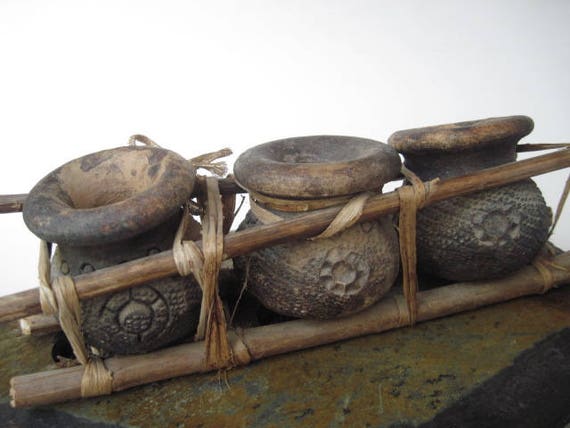This close-up photograph features three intricately designed pots with a rich brown hue. Each pot showcases indented circular symbols, with a common design element of a central circle. The two pots on the left have central circles encircled by six small semicircles, while the third pot features a central circle with six equidistant gouges around it. The tops of the pots flare outward and have a bronze tone, adding a striking contrast. 

These pots are secured in a rustic holder made of four wooden sticks, two in the front and two in the back, tied together with brown twine or possibly plant material. The twine stretches in between each pot and presumably binds to the back sticks, ensuring stability. The entire assembly rests on what appears to be a weathered brown stone or perhaps an old tree stump, adding to the ancient, artisanal feel of the image. The background is a white wall, with the right corner cast in shadow, further highlighting the earthy tones and intricate details of the pots and their holder.